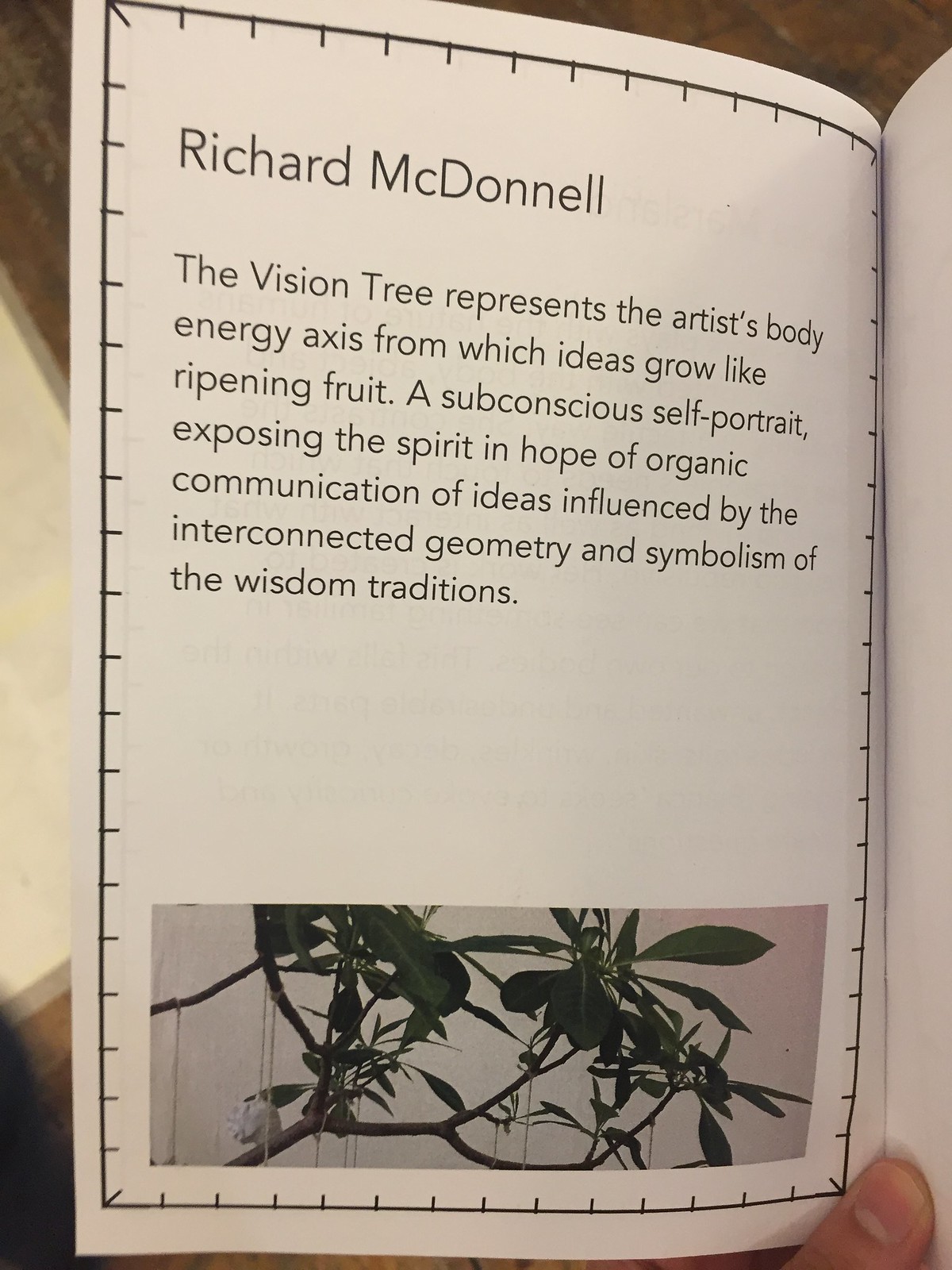This photo captures an open page of a book with a clearly defined black border and fine lines extending from its edges. The prominent title "Richard Macdonald" introduces the content which delves into the concept of the vision tree. The text poetically describes the vision tree as a metaphor for the artist's body, a source of energy from which ideas flourish like ripening fruit. It is depicted as a subconscious self-portrait revealing the spirit and hope of organic communication of ideas, deeply influenced by the interconnected geometry and symbolism inherent in wisdom traditions. At the bottom of the page, there's an illustration of a branch adorned with capsule-shaped green leaves and a singular white rose, accentuating the organic theme. The background of the entire scene is a plain white, providing a clean canvas for the detailed imagery and text. A person's thumb is visible at the bottom center-right, firmly holding the page open, ensuring the viewer's focus remains undisturbed on the intricate details and profound message conveyed.